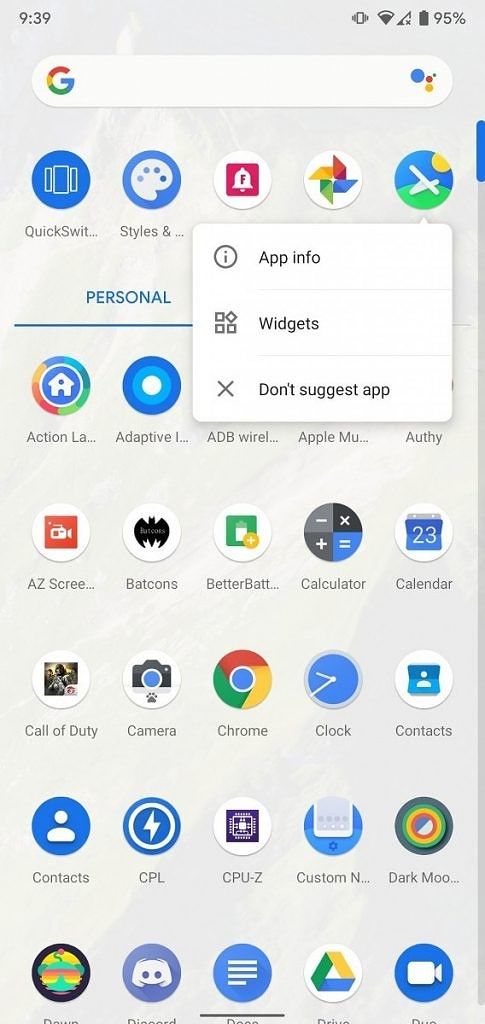Screenshot of a mobile device displaying the Google app interface at 9:39 AM with a full battery at 95%. The device has cellular service but lacks a Wi-Fi connection, indicated by an 'X' over the Wi-Fi symbol. The search bar features the multicolored 'G' logo of Google. Below the search bar, multiple apps are visible, including Quick Switch, Styles, Action Launcher, Adaptive, Apple Music, Authy, AZ Screen Recorder, Batcon, Calendar, Call of Duty, Chrome, Clock, Contacts, Custom Dark Mode, Discord, Duo, among others. The screen also shows an option menu with "App info," "Widgets," and "Don't suggest app," along with an option to close (X) the menu. The screenshot doesn't clearly indicate whether the device is a phone or a tablet.